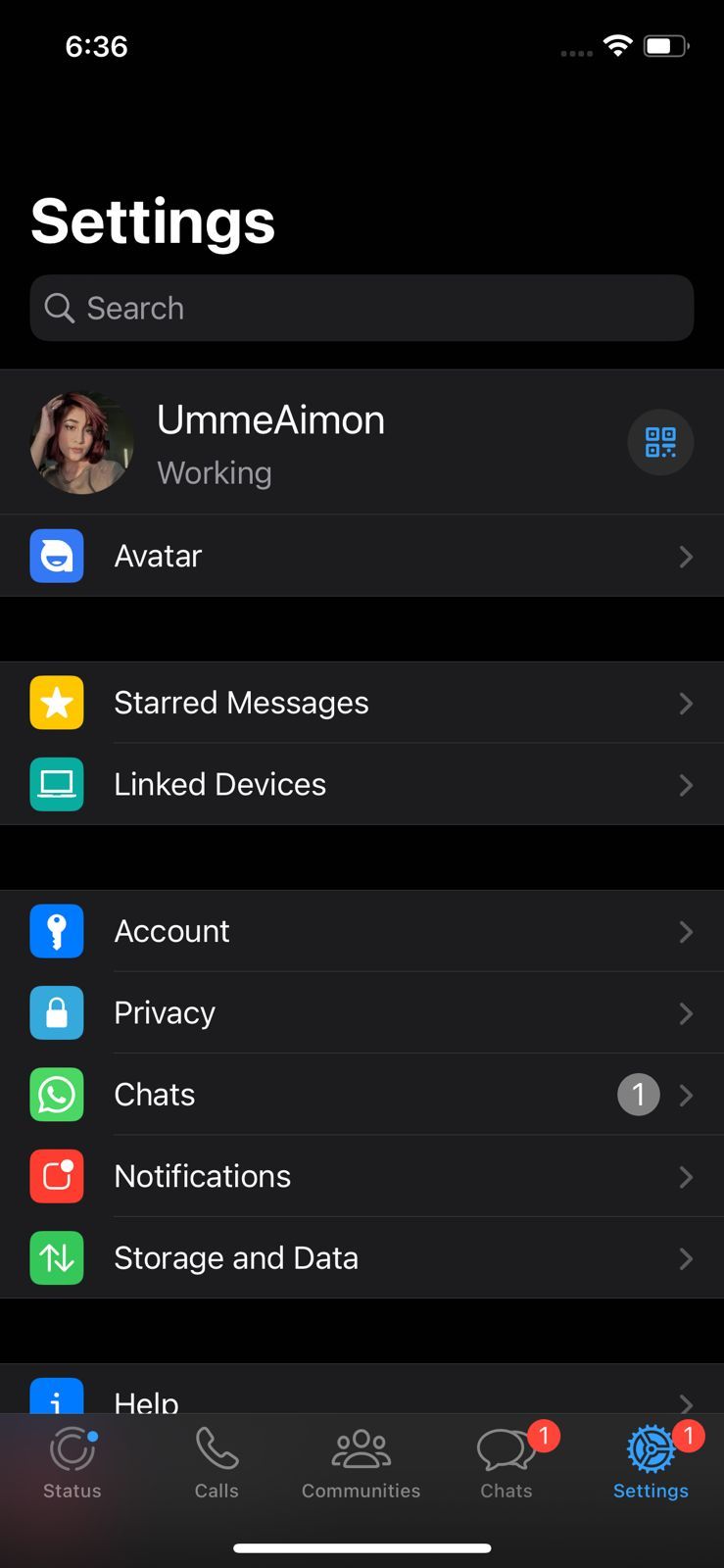A screenshot of a smartphone's settings section features a prominent black background. The time displayed is 6:36, and four minimalistic navigation dots can be seen lined up along the bottom right corner of the screen. The Wi-Fi signal icon indicates a full connection, and the battery status is approximately 70%. The word "Settings" is displayed at the top in thick, bold, white font.

Below the header is a search field with a magnifying glass icon and the placeholder text "Search." Following this, the name "Ummeaimon," with the 'U' and 'A' capitalized, is displayed next to a circular illustration of a woman, labeled "Working."

Further down, an A-shaped logo in a blue square is labeled "Avatar." Thereafter, there is a black bar sectioning off the next area, which features two gray sections: one with a white star on a yellow field labeled "Starred Messages," and the other with a white laptop on a green square labeled "Linked Devices."

Another black line separates this from five additional sections. These include: 
1. "Account" with a key icon on a blue square,
2. "Privacy" with a lock icon on a lighter blue square,
3. "Chat" with a text bubble icon resembling WhatsApp on a green square, which has a small gray circle on the right indicating the number one,
4. "Storage and Data" with a square bearing a dot on red,
5. "Help" with a question mark icon.

Lastly, the navigation bar at the bottom includes status calls, communities, chats, and settings options. Both the chats and settings icons have a red circle with the number one inside, indicating new notifications.